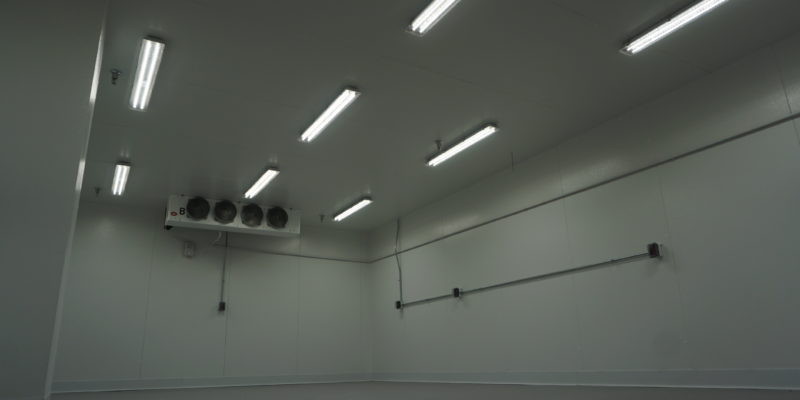The image depicts a stark, empty room characterized by its white walls and ceiling. The room is illuminated by an array of track lighting, with three fixtures positioned at the back, three in the middle, and another set of three directly overhead. Of the latter set, only two lights are visible, while the third remains obscured. 

At the back of the room, an electrical cord descends, suggestive of a close installation to the four fans whose square white boxes feature a central black circle, presumably the fan blades. On the right side of the room, a strip runs horizontally, housing three electrical outlets evenly spaced. The walls are segmented into square white panels, adding a grid-like texture to the space. 

Notable among the light fixtures, particularly the two on the left side, are sprinkler systems attached near them. In the section of the ceiling adjacent to the middle aisle, the next row of lights features two sprinklers, each positioned beside a light fixture. This detail suggests a robust fire safety system integrated into the room's design.